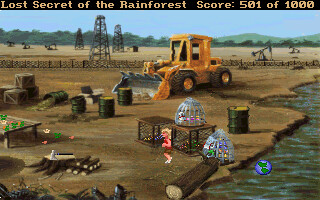A tiny square video game screenshot titled "Lost Secret of the Rainforest" is displayed with a score of 501 out of 1,000 at the top. The scene depicts a bustling construction site dominated by a giant yellow backhoe, actively scooping dirt in the center. Scattered around are numerous black and green oil barrels, some of which have spilled their contents. Metal cages and piles of logs and wooden crates litter the area near the right side. In the forefront, a cartoon-like character with blonde hair, pink arms and legs, a red shirt, brown shorts, and yellow shoes walks, seemingly sneaking in front of the cages. Towards the right corner, a muddied waterway contains a floating blue ball. The background is marked by oil derricks and a large fence, with green trees and hilly terrain further back, completing the scene.